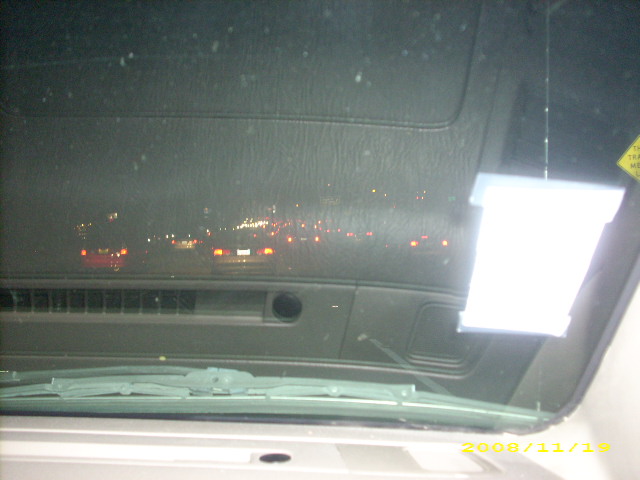This image is a color snapshot captured from the passenger seat of a vehicle at night. The lower portion of the photograph displays a reflection of the dashboard, including the air conditioning vents. The vehicle's actual dashboard is illuminated in the shot, with faint squiggly textures visible from the leather material. A yellow date stamp in the bottom right corner indicates "2008-11-19." A bright, square-shaped glare occupies the center-right section of the image, partially obscuring the view. Through the windshield, the highway scene reveals several vehicles with illuminated taillights and headlights, highlighting the bustling activity. A windshield wiper is also visible. In the upper right above the brilliant glare, a corner of a yellow street sign with some text comes into view, adding context to the nighttime environment.